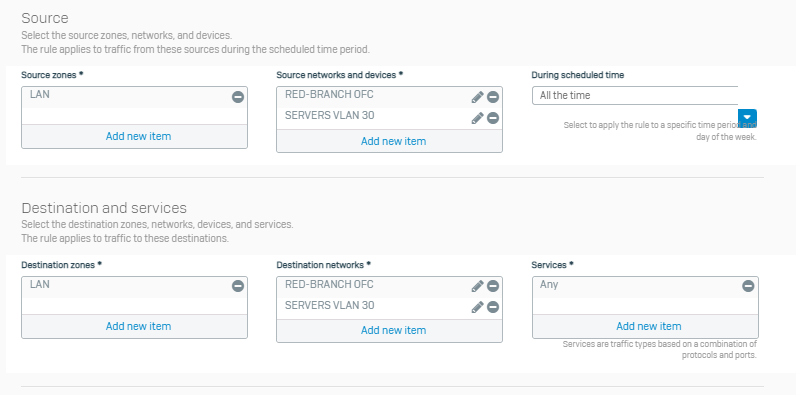The image displays a user interface for configuring network traffic rules, starting with the "Source" section at the top left corner, highlighted in larger text. This section involves selecting source zones, networks, and devices. Below this, it explains that the rules will apply to traffic from these sources during scheduled time periods.

Two main panels are present: 

1. **Source Zones**
   - A top label marked with an asterisk reading "Source Zones".
   - The panel lists items in alternating gray and white rows: "LAN" (with an option to add new items in blue) and includes a minus sign for deletion.

2. **Source Networks and Devices**
   - Similarly labeled with an asterisk and titled "Source Networks and Devices".
   - Inside the box, items include "Red Branch OFC" and "Servers VLAN 30", each with options to edit (pencil icon) or delete (minus icon). An option to add new items is also present.

Below these panels is a drop-down menu titled "During Scheduled Time", set to "All the time," indicating the timing rules for applying these settings.

The next section, "Destination," includes:

- **Destination Zones**
  - Titled "Destination Zones", with listed items like "LAN" which can be deleted or added.
- **Destination Networks**
  - Lists options such as "Red Branch OFC" and "Servers VLAN 30" with edit and delete functionalities.
  
Lastly, the "Services" category defaults to "Any" but allows for addition or removal of specific services.

In summary, this interface enables detailed configuration of network traffic rules through a series of selectable and editable source and destination parameters, all with timing customization.